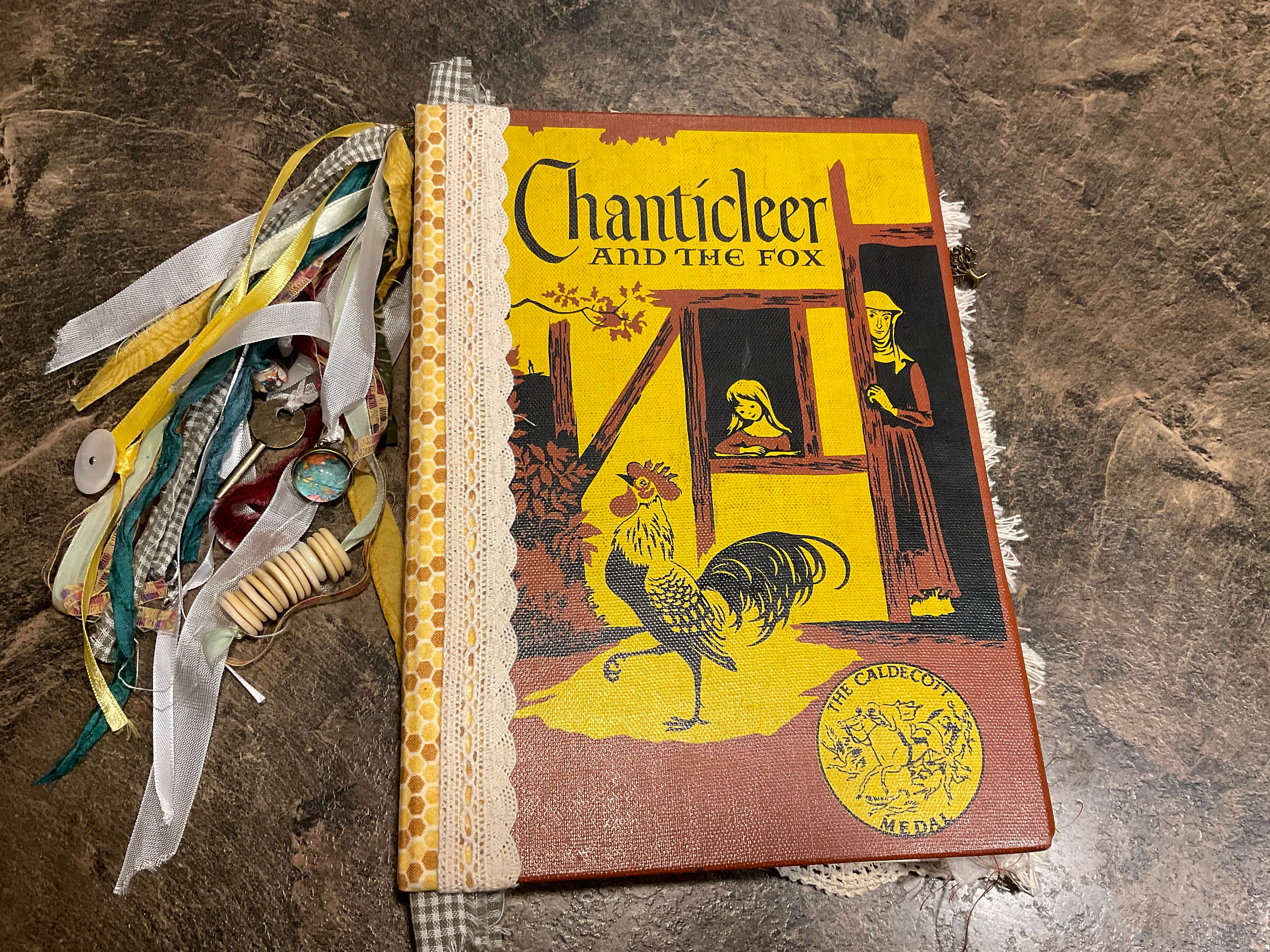This is a horizontally aligned rectangular image featuring an old, yellow-covered book resting on a textured, brown stone surface. The book, titled "Chanticleer and the Fox," prominently displays its title in black text at the top center. Below the title, there is an illustrated scene depicting a little girl looking out of a window, while her mother peers around a doorway at a rooster walking to the left. Both characters are dressed in maroon outfits. The book's cover features a circular emblem in the bottom right corner, which is the Caldecott Medal, signifying its prestigious status in children's literature. The spine of the book is adorned with a hexagonal pattern in alternating light and dark brown shades, outlined in white, complemented by white lace running along the left edge down to the right. Various decorative objects, including ribbons, buttons, and keys, hang from the top of the spine, adding an intricate and nostalgic touch to the overall presentation.